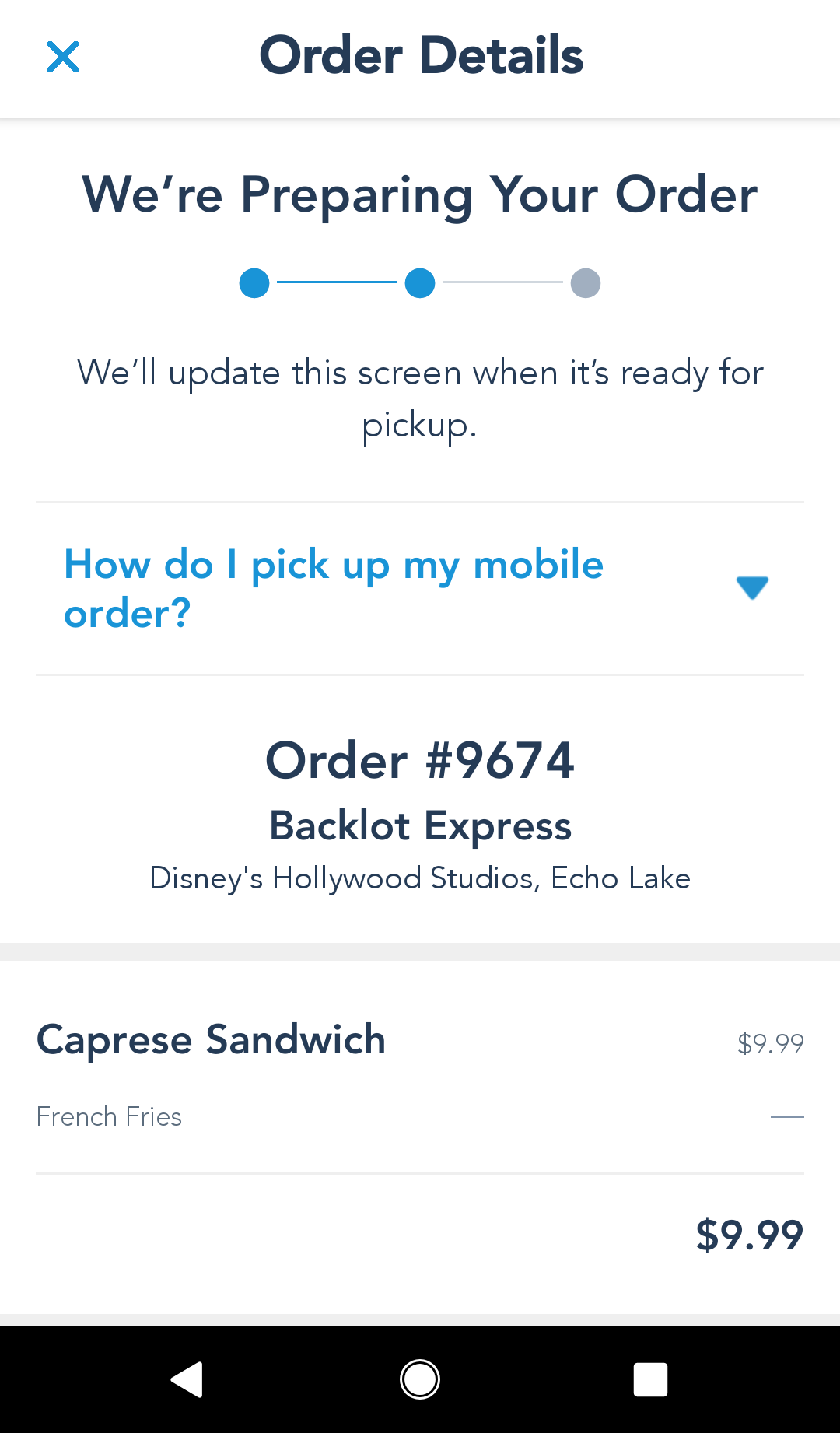This image features a predominantly white background with a prominent blue "X" and black text detailing order information. At the top, the text reads, "We're preparing your order," followed by three circles—two blue and one gray, indicating the order's status. Below this, it states, "We'll update this screen when it's ready for pickup."

Further down, there is a section with expandable text, indicated by "How do I pick up my mobile order?" in blue with a down arrow next to it. Beneath this section, the order specifics are listed: Order number 9674 from Backlot Express located in Disney's Hollywood Studios, Echo Lake. The items ordered include a Caprese Sandwich priced at $9.99 and French Fries, also priced at $9.99.

At the bottom of the image, there is a black footer featuring white icons: an arrow pointing left inside a circle and a square.